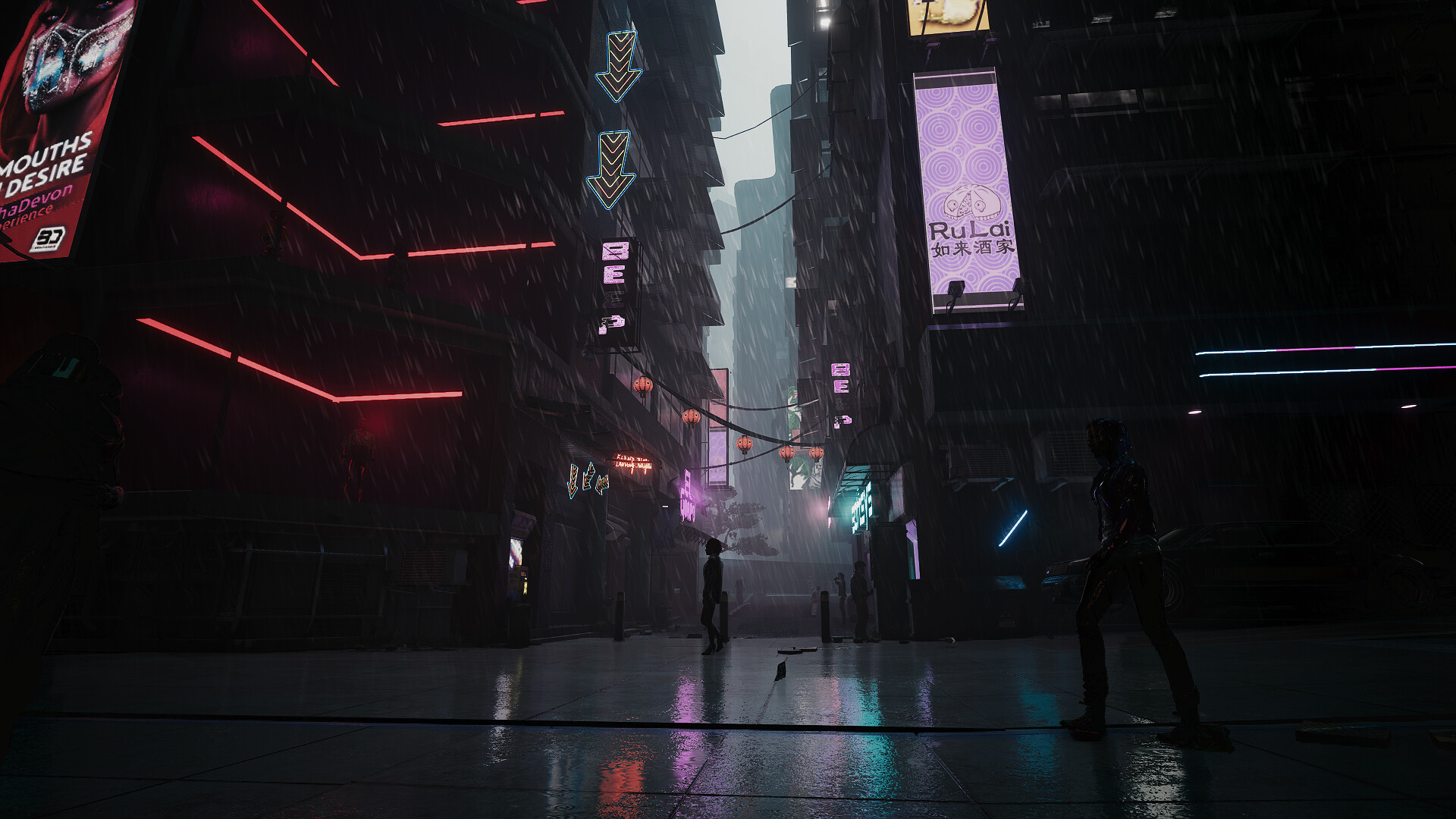The image captures a screenshot from a visually striking video game featuring a dystopian, Blade Runner-esque downtown scene. A narrow alleyway is flanked by towering skyscrapers, their dark facades illuminated by vivid neon lights. The ground is wet and reflective from the rain, enhancing the scene's atmospheric mood. In the foreground, a courtyard appears, with shadowy silhouettes of people walking through the slick, concrete surface. The left building is adorned with red neon arrows and a prominent billboard in the top corner, while the right building features a purple neon sign and a smaller yellow sign. Japanese lanterns strung between the structures glow softly, adding to the cyberpunk aesthetic. The blend of modern architecture, neon brilliance, and rainy ambiance evokes a sense of immersion into a futuristic world.